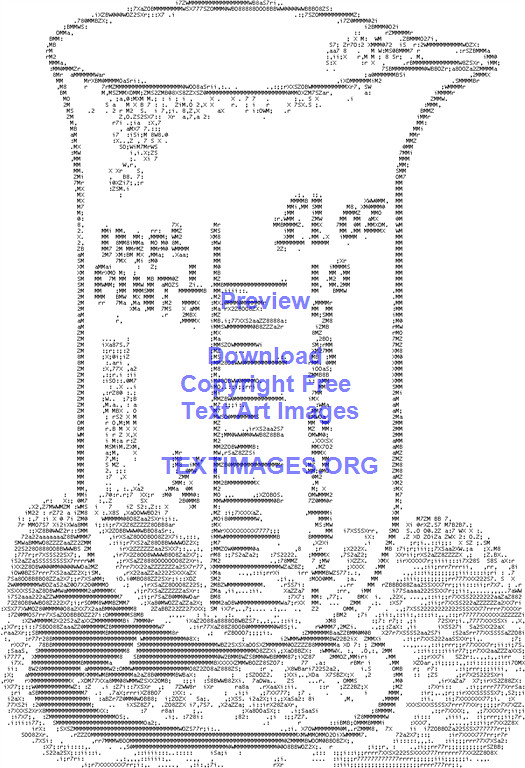This image depicts a digitally created, pixelated outline of a measuring cup with a spout facing right, rendered in various shades of gray, white, and royal blue. The measuring cup features both Imperial and fluid ounce measurements. On one side, it reads "IMPL pint half," and on the other side, it marks fluid ounces from 10 down to 1. The cup sits against a background filled with numerous small numbers. Overlaid on the image in blue text are the words "Preview Download Copyright Free Text Art Images" and "textimages.org," indicating that this is a free-text art image available for download. The overall setup and style suggest a software-created digital artwork.